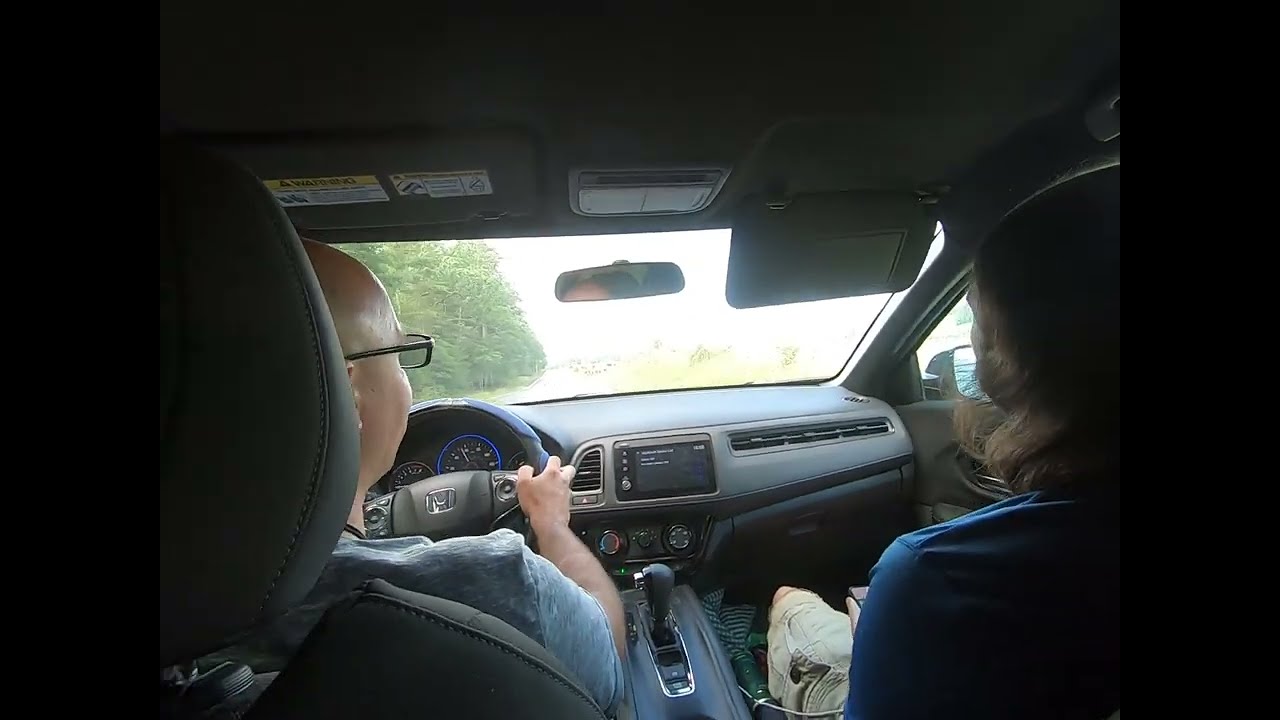The photograph captures the interior of a Honda sedan from the perspective of the backseat. In the driver's seat is a middle-aged, bald man with glasses, wearing a grayish-blue t-shirt. His hands are on the steering wheel, and the car's interior appears predominantly gray. To the right, in the passenger seat, sits a person with shoulder-length brown hair, donned in a blue shirt and khaki cargo shorts. The passenger's sun visor is flipped down. The view through the windshield is bright and mostly white, making it difficult to discern details, although faint outlines of a tree and some foliage are visible. The dashboard has a light bluish hue, and a rearview mirror is mounted on the windshield. The image provides a cozy look into a ride, with the driver seeming to be navigating the vehicle, evident from his focused grip on the steering wheel.